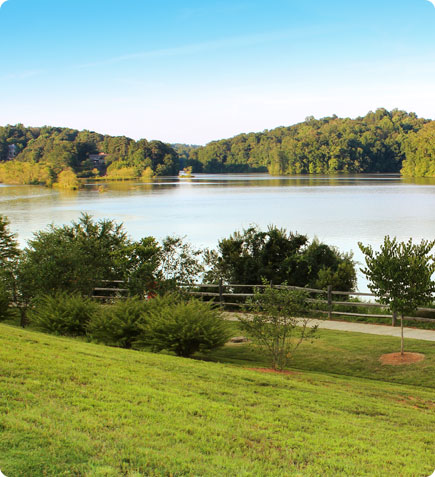This image depicts an expansive, serene outdoor setting centered around a large lake, likely a lake, surrounded by an array of trees that envelop the entire scene in lush greenery. The clear, blue sky above stretches without a hint of clouds, adding to the tranquility of the setting. In the foreground, a grassy hillside slopes gently downwards, dotted with smaller trees, each surrounded by spots of mulch or dirt. A wooden split rail fence runs parallel to a concrete walking path that encircles the lake, offering a scenic route for strolls. The predominant colors in the photo are blue, green, and white, accented by the earthy tones of brown from the fence and mulch, and gray from the path. The image conveys a peaceful, natural environment with no additional objects or text, capturing a pure, idyllic lakeside view.